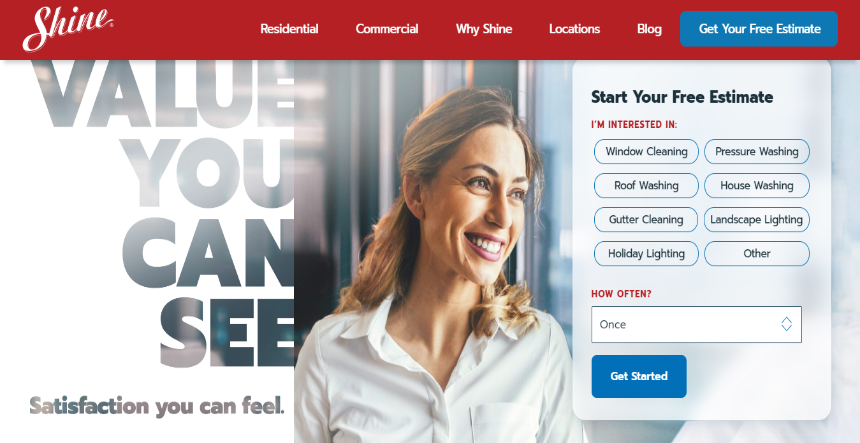Promotional Banner for Shine Cleaning and Maintenance Services

The top section of the promotional banner features a vibrant red background with the Shine logo displayed in white on the left. Navigation links—Residential, Commercial, Why Shine, Locations, Blog, and Get Your Free Estimate—are prominently highlighted, with the "Get Your Free Estimate" link standing out as a large blue button.

Dominating the left side of the banner, in bold and large typography, is the phrase "Value You Can See," followed by "Satisfaction You Can Feel" in slightly smaller letters. Beneath this text is an image of a woman smiling as she gazes out of a window, embodying a sense of contentment and cleanliness.

Below the woman's image, a call-to-action for "Start Your Free Estimate" is presented, guiding users to a form. The form includes checkboxes for various services such as window cleaning, pressure washing, roof washing, house washing, gutter cleaning, landscape lighting, holiday lighting, and an option for other services. Drop-down menus or labels are available for selecting the frequency of service. The form concludes with a blue "Get Started" button.

The overall design is professional and meticulously structured to emphasize Shine's comprehensive range of services, effectively urging potential customers to take advantage of the complimentary estimate offer.